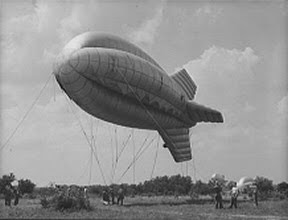This vintage black-and-white photograph showcases a large, helium-filled blimp floating in the air against a cloudy sky. The blimp, resembling a fully inflated balloon, features concentric circles running from its nose to its tail. It is equipped with three visible fins – one on top, one on the bottom, and one on the side – with a possible fourth fin obscured from view. Numerous lines tether the blimp to the ground, some anchored to the earth and others held by an estimated nine people, although a few could be partially hidden by background elements. Groups of individuals stand on a grassy field, observing the blimp, with trees and the faint outline of a building in the distant background. The photograph, despite its age, captures the enormity and intricacies of the blimp, making it a detailed and fascinating historical record.